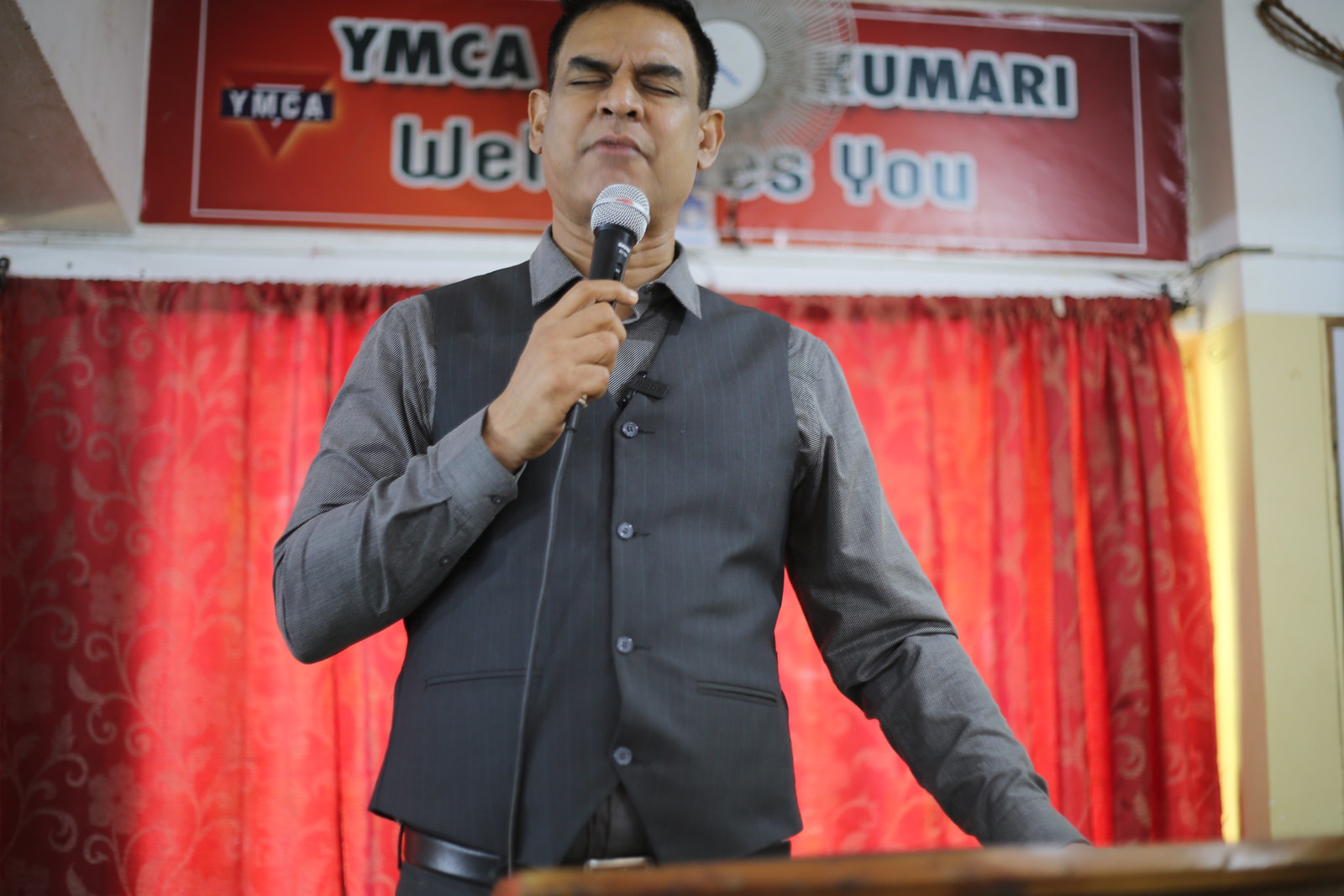The photograph captures a moment inside an auditorium where an Indian man stands at a wooden podium. He is holding a wired microphone and appears to be giving a heartfelt speech, as conveyed by his closed eyes and furrowed brows, suggesting deep emotion or prayer. He is dressed in a gray long-sleeved collared shirt underneath a black pinstriped vest, complemented by dark pants and a black belt. Behind him, a tall red curtain hangs against a backdrop of white and yellow walls. Above the curtain, a large red sign with black font and a white border reads "YMCA Kumari welcomes you," accompanied by a small YMCA logo and a clock positioned between the "YMCA" and "Kumari." A rotating fan is also visible in the background.